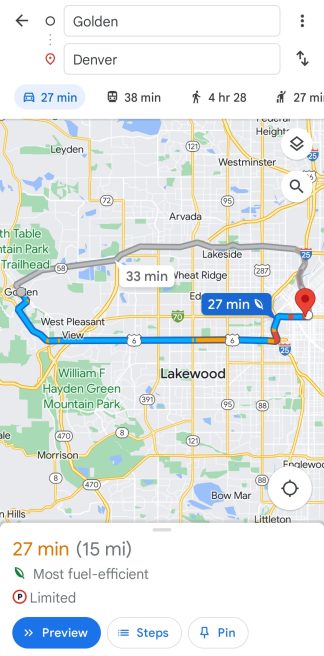This screenshot showcases a mobile application interface designed to provide detailed driving directions between two locations. The primary visual element is a map illustrating the requested route. The background is a standard white, while text elements are in black for readability. At the top of the screen, the starting location is listed as Golden, Colorado, and the destination as Denver, Colorado.

The app presents multiple travel options:
- A 27-minute drive, which appears to be the fastest and currently selected route.
- A bus journey taking 38 minutes.
- A walking route estimated at 4 hours and 28 minutes.
- A taxi or ride-sharing option that would also take 27 minutes.
- An alternative driving route lasting 33 minutes.

No additional images are present aside from the map and the depicted route options.